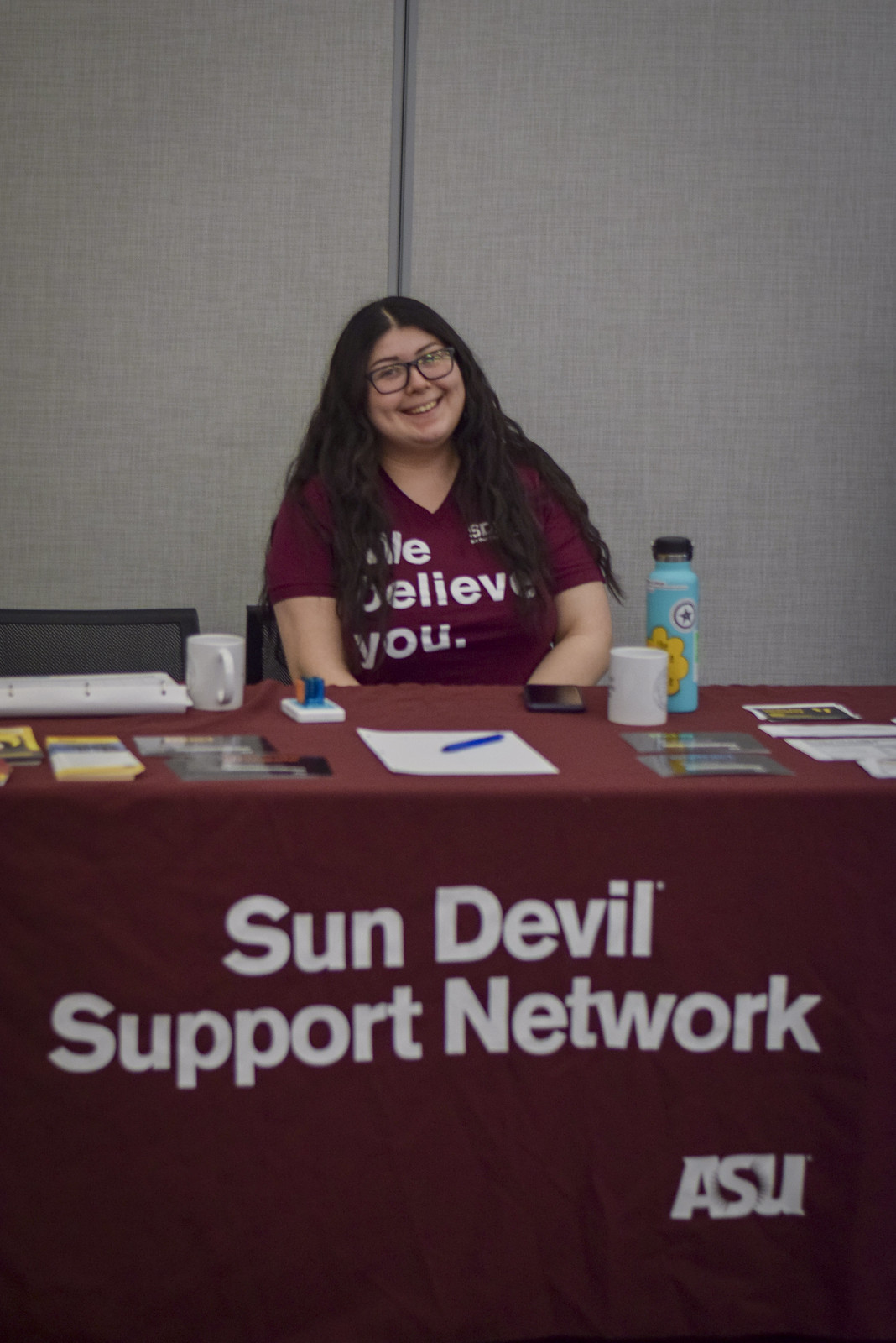The image captures a young Hispanic woman, likely in her 20s, sitting cheerfully at a table inside what appears to be a conference hall. She has long, wavy, dark brown hair cascading past her shoulders and wears glasses. Her maroon, V-neck t-shirt emblazoned with "We Believe You" matches the tablecloth on the display in front of her, which reads "Sun Devil Support Network, ASU." 

The table is adorned with a variety of items: a light blue water bottle with a yellow flower, two white coffee mugs, a smartphone, a piece of paper accompanied by a blue pen, and numerous brochures or pamphlets. An empty chair is positioned nearby, and the background features a gray wall. The woman’s bright smile radiates warmth and invitation, enhancing the welcoming atmosphere of the setting.